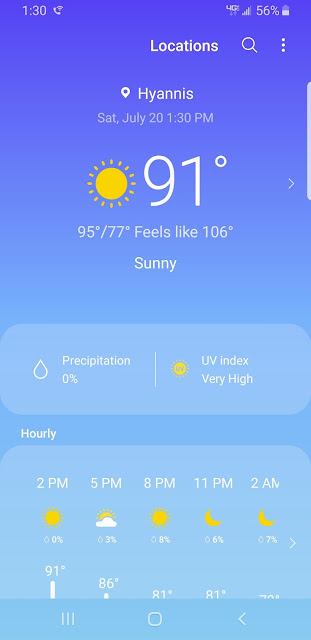In this image, a weather application is displayed on a smartphone screen against a vibrant blue background, which transitions from deep blue at the top half to light blue at the bottom half. At the top of the screen, the status bar is visible with several white icons: the time on the top left, a Wi-Fi calling icon, a 4G network icon, and a battery icon showing 56% on the top right.

The application is set to the location "Hyannis" and features a search bar and options menu. The current weather details for Hyannis on Saturday, July 20 at 1:00 p.m. indicate a temperature of 91°F, with a high of 95°F and a low of 75°F. The sky is depicted by a yellow sun icon, symbolizing sunny weather. A note indicates that it feels like an extreme 160°F. Below this, further details show 0% precipitation and a UV index that is very high, also highlighted by a yellow sun icon.

The bottom section of the application provides an hourly weather forecast:
- At 2:00 p.m., the temperature remains 91°F.
- By 5:00 p.m., the temperature drops to 86°F with a 3% chance of precipitation.
- At 8:00 p.m., the temperature further decreases to 81°F with an 8% chance of precipitation.
- At 11:00 p.m., the temperature remains 81°F with a 6% chance of precipitation.
- By 2:00 a.m., the precipitation increases to 7% and the temperature is in the 70-degree range.